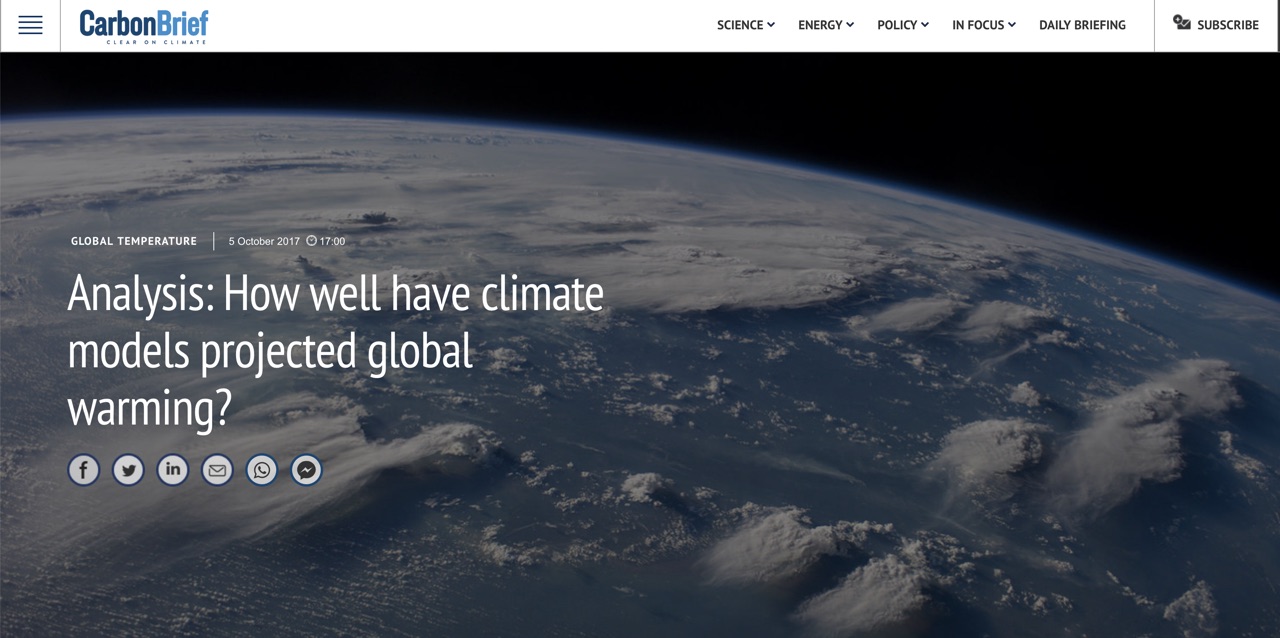Here is a cleaned-up and detailed caption for the image described:

---

Desktop application screenshot for the "Carbon Brief" platform. In the top left corner, the "Carbon Brief" logo is displayed, comprising four navy blue horizontal lines stacked on top of each other. To the left of the logo are various settings options. The logo features the word "Carbon" in navy blue and "Brief" in a lighter blue color. Below the logo, in small font, the phrase "Clear on Climate" is written.

Across the top of the interface are several dropdown menus labeled "Science", "Energy", "Policy", and "Focus Daily Briefing". On the extreme top right, there is a "Subscribe" button.

Dominating the background is a stunning image of Earth as seen from space, enveloped by the blackness of the cosmos. Superimposed over this image is the text "Global Temperature", with a timestamp reading "October 5, 2017, 17:00 (5:00 p.m.)".

Below this, a headline reads "Analysis: How well have climate models projected global warming?" To the right of this headline are shortcut icons for sharing via Facebook, Twitter, LinkedIn, Gmail, WhatsApp, and Facebook Messenger.

---

This detailed caption encapsulates the various elements and context provided in the image.